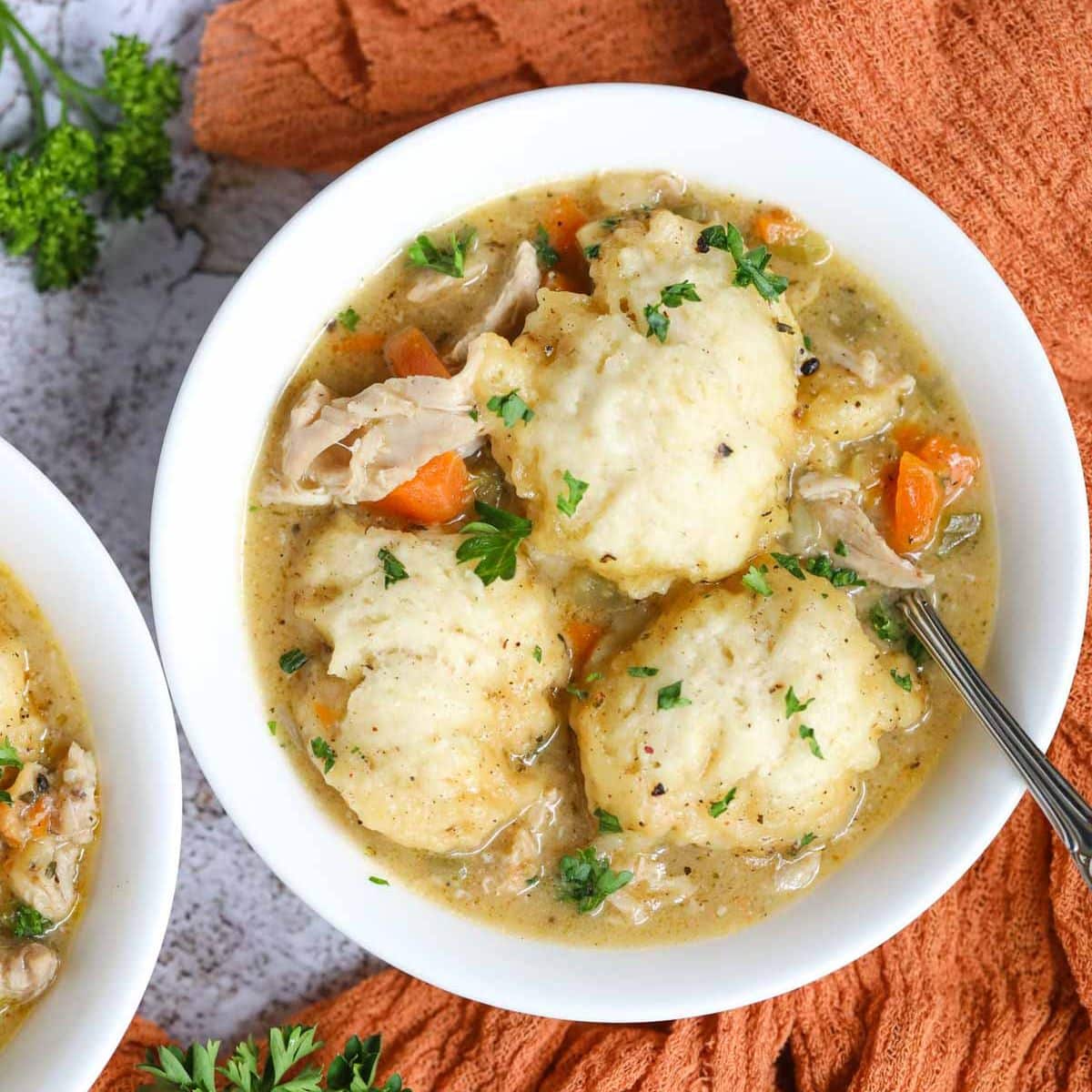The image captures a close-up of a meal featuring two bowls of soup on a table. The primary bowl, prominently in focus, contains a hearty chicken soup with visible chunks of lean meat, sliced carrots, and garnished with parsley. Floating in the light brown broth are three substantial dollops of what appear to be mashed potatoes, though they could be semolina dumplings. The bowl is situated on a surface that is partly covered with an orange cloth, adding a warm contrast to the scene. A spoon is seen diving into the soup, poised to scoop up its contents, though no hand is visible. To the left, there is a partial view of another bowl of soup, hinting at a similar composition but not fully visible to confirm. The detailed composition of the soup, with its vibrant vegetables, meat, and sizable dumplings or mashed potatoes, forms the central focus of this inviting meal setting.